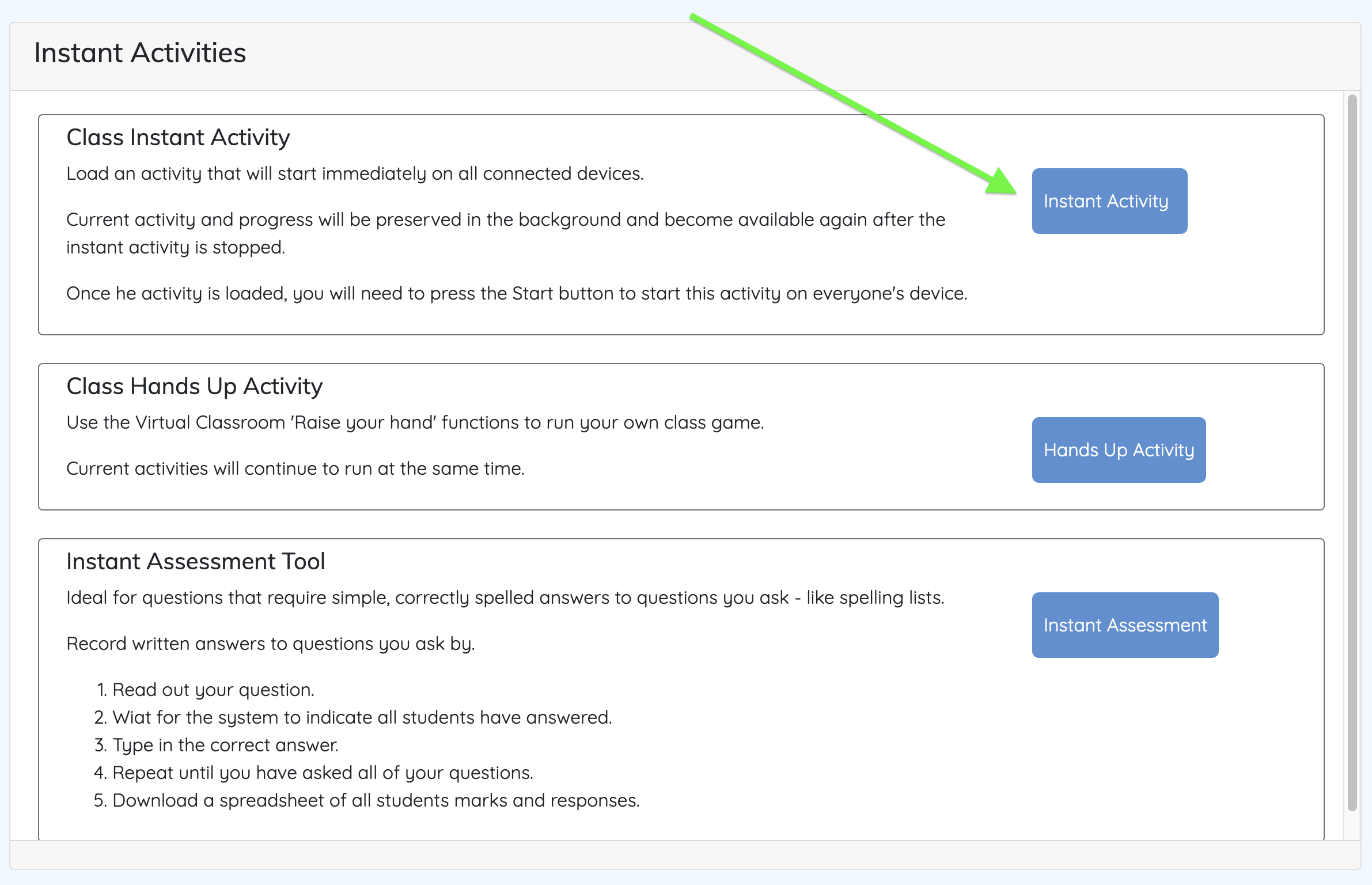The image features a screenshot highlighting a section titled "Instant Activities" situated on the upper left-hand side in black font. The words "Instant Activities" are capitalized with the initial letters "I" and "A" prominently standing out.

A green arrow directs attention towards a prominent blue button labeled "Instant Activity" in white font. This button is integral to the three distinct sections outlined in the screenshot.

Each section is dedicated to a different type of "Instant Activity" and is accompanied by a corresponding blue button labeled "Instant Activity" on the right-hand side. 

The first section is labeled "Class Instant Activity." This section explains that you can load an activity that will immediately start on all connected devices. The instructions detail that any current activity and its progress will be preserved in the background, allowing it to be resumed once the instant activity is stopped. Moreover, it specifies that after the instant activity is loaded, you must press the "start" button to activate it on everyone's device.